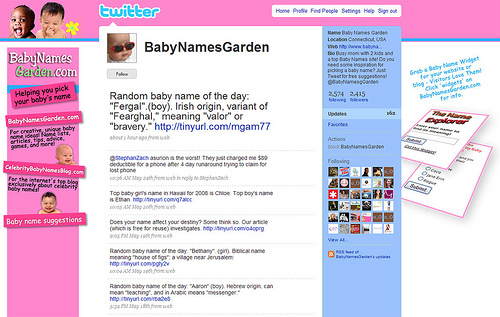The webpage, clearly designed with a youthful and playful vibe, features a vibrant and engaging layout aimed at parents searching for baby names. In the top left corner, an endearing image captures an African American baby and an Asian baby, both with short black hair, smiling and laughing joyfully. The Asian baby also has his hand playfully touching his face.

On the right side of the page, a cheerful yellow flower with a green center can be seen. Adjacent to it, a playful, bubbled text reads "Twitter" in blue letters. Just beside this, a mid-gray rectangle houses clickable blue text buttons for easy navigation, labeled: Home, Profile, Find People, Settings, Help, and Sign Out.

Center stage, beneath the Twitter section, a close-up photograph of a baby wearing trendy red sunglasses with black lenses draws attention. To the right of this image, the bold text "Baby Names Garden" is prominently displayed. Below the baby’s photo, a mid-gray box with black text invites users to "Follow."

Next, a highlighted feature presents the "Random Baby Name of the Day," showcasing the name "Frugal Boy," which is noted to have Irish origins and is a variant of "Fearghal," meaning "valor" or "bravery." A tiny URL link (http://tinyurl.com//mgam77) provides a shortcut, followed by several Twitter strings.

On the left side, the website address "babynamesgarden.com" is displayed. Above a blue line, a tilted hot pink rectangle with black text reads, "Helping you pick your baby's name." Another rectangle, tilted to the right and also hot pink, displays the site’s name "babynamegarden.com" in white text. Additionally, black text beneath it highlights the website’s offerings: "For creative unique baby name ideas, name lists, articles, tips, advice, games, and more."

Further down, a slanted rectangle pointing right reads "celebritybabynames.com," indicating a top blog focused exclusively on celebrity baby names. Lastly, a hot pink rectangle, slightly angled upwards, features a picture of a baby similar to the one previously shown. It caps off with the text "babynamesuggestions" in white.